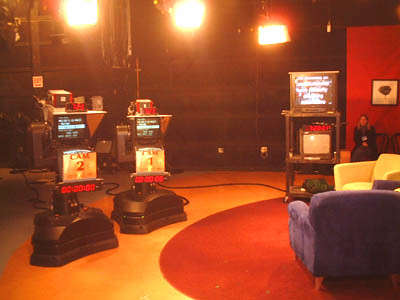This detailed photograph appears to be the set of a TV program, possibly a talk show or a news station. The studio is well-lit with three prominent stage lights hanging from the ceiling, which illuminate the set. Front and center, there are two chairs – one blue with a pillow and one yellowish, likely a couch – positioned catty-corner to each other on a large, round red rug. The chairs are complemented by a striking floor design featuring crescents.

In the backdrop, a woman is seated on one of the two wooden-backed chairs situated near a red wall that features a painting, possibly of a tree. Nearby, an exit sign and various cords indicate the presence of a lot of equipment. The set is populated with several cameras, including two labeled CAM-1 and CAM-2. There's also a teleprompter with an old-school TV monitor beneath it, displaying white text which is not entirely legible, suggesting it's being used to guide on-screen talent.

The floor is a distinctive brown color, contributing to the overall warm and professional ambiance of the studio. Details like the equipment cords running across the floor and the monologue on the TV monitor, positioned on a tall stand, emphasize the dynamic and functional environment of the recording studio.